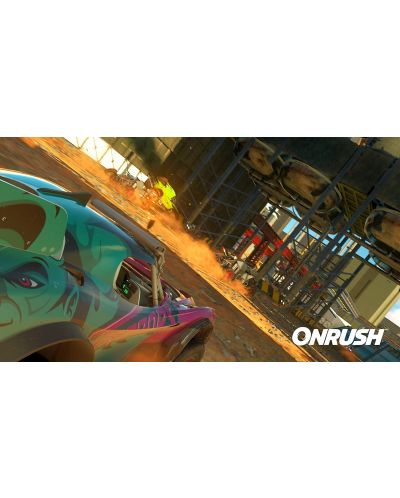The image depicts a vibrant, highly detailed, computer-generated race car angled about 45 degrees to the right. The car, reminiscent of those seen only in video games, features a striking blue and purple color scheme with teal and darker blue accents. Only the rear half of the car is visible, revealing a stylized face with an eye and what appears to be a partial smile on the back. This futuristic vehicle is situated in an industrial environment characterized by red girders, large metal structures, and yellow and black hazard barriers. The background includes an industrial building with windows letting in sunlight, casting brown dust in the air, and revealing a distant cityscape with a blue sky. In the lower right-hand corner of the image, the word "Onrush" is prominently displayed in white, all-capital letters. Additionally, a peculiar bright yellow object, possibly resembling a tiny explosion, is visible in the upper middle portion of the scene.